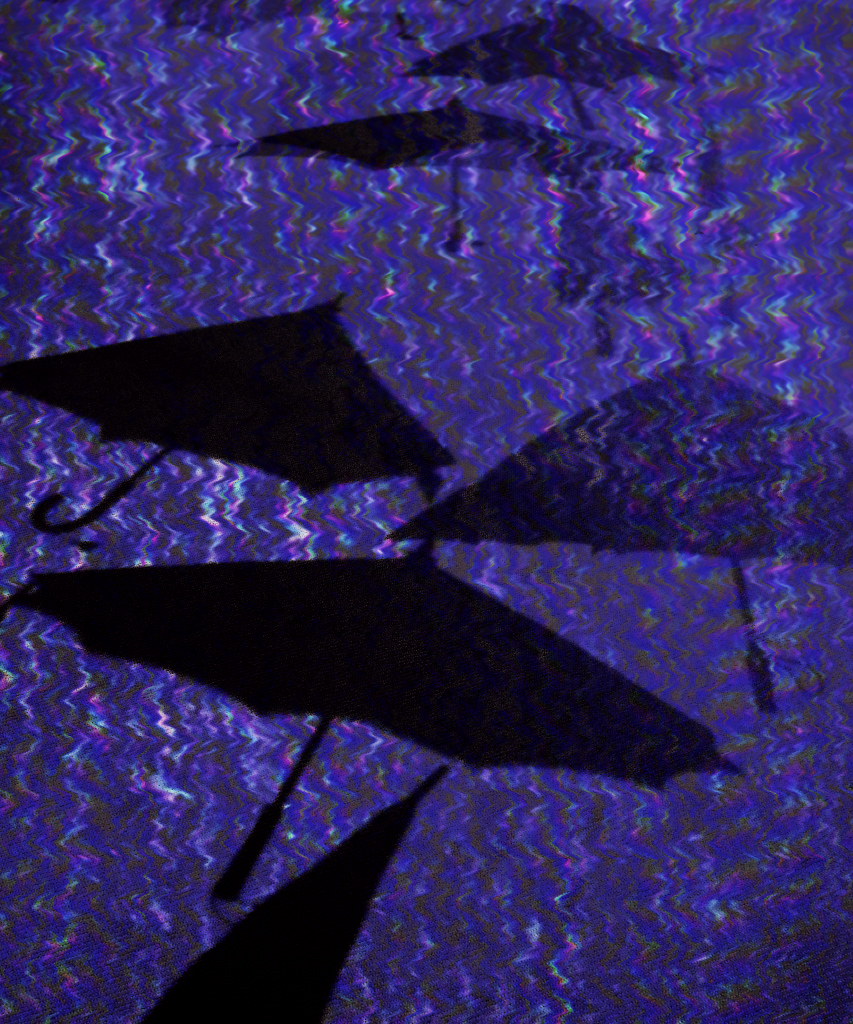The image depicts a highly detailed, hand-painted artwork that conveys an otherworldly, almost underwater scene. The background is composed of a wavy, rippling blue pattern, enhanced with vertical squiggly lines in hues of white, pink, purple, and black, creating a holographic or prismatic effect. The scene features at least six black silhouettes of umbrellas, varying in shape and state. Most are open, showing their dark, shadowy forms prominently against the vibrant background, while one at the bottom appears to be closed, presenting a distinct pyramid cone shape. These umbrellas, seemingly floating and casting shadows, have handles in diverse styles—some straight and others curved, resembling the letter 'J.' The umbrellas appear to be suspended in the center, creating an illusion of motion and surrealism, further emphasized by the absence of any visible support. The overall effect is a mesmerizing blend of colors and shapes, producing a dynamic, hologram-like visual experience.